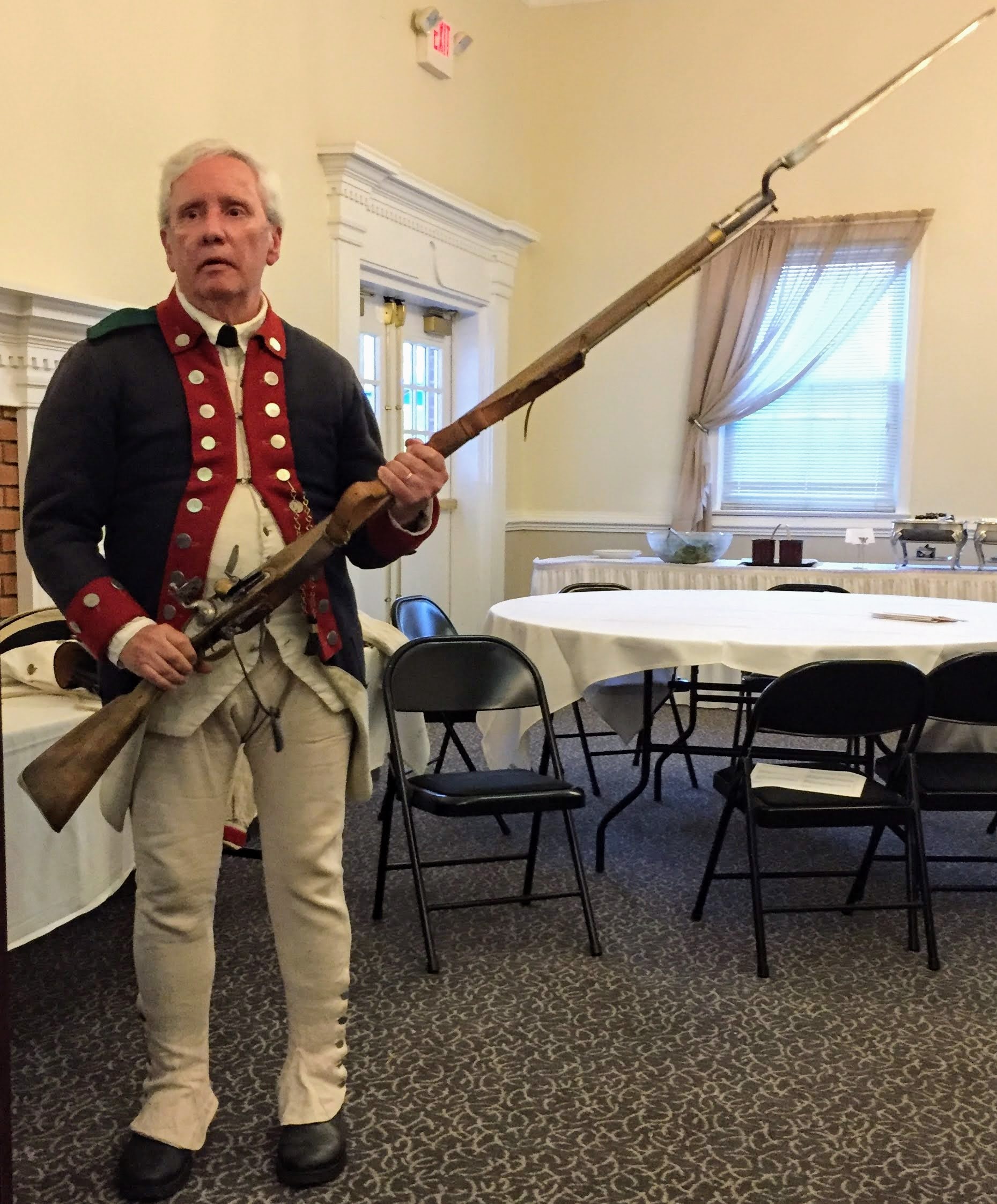In this photo, an elderly man is posing in a detailed revolutionary-era uniform, likely for a historical reenactment. His ensemble includes a long, black coat adorned with red accents along the collar, down the front, and around the wrists, all fastened with silver buttons. Beneath the coat, he wears a beige vest and pants, the latter being somewhat bulky at the crotch and buttoned down to the black shoes at the ankles. He holds a substantial, long musket with a silver bayonet attached to the wooden barrel; his right hand grips the area near the trigger while his left steadies the gun near the bottom of the barrel.

The setting appears to be a dining hall, characterized by round tables draped with white linens and surrounded by black folding chairs. To the right of the man, there is a round table with a white tablecloth, and further back, a long table holding silver food containers and glasses, suggesting a buffet setup. Behind him, there's a door to the left and a window to the right, completing the nuanced indoor scene.